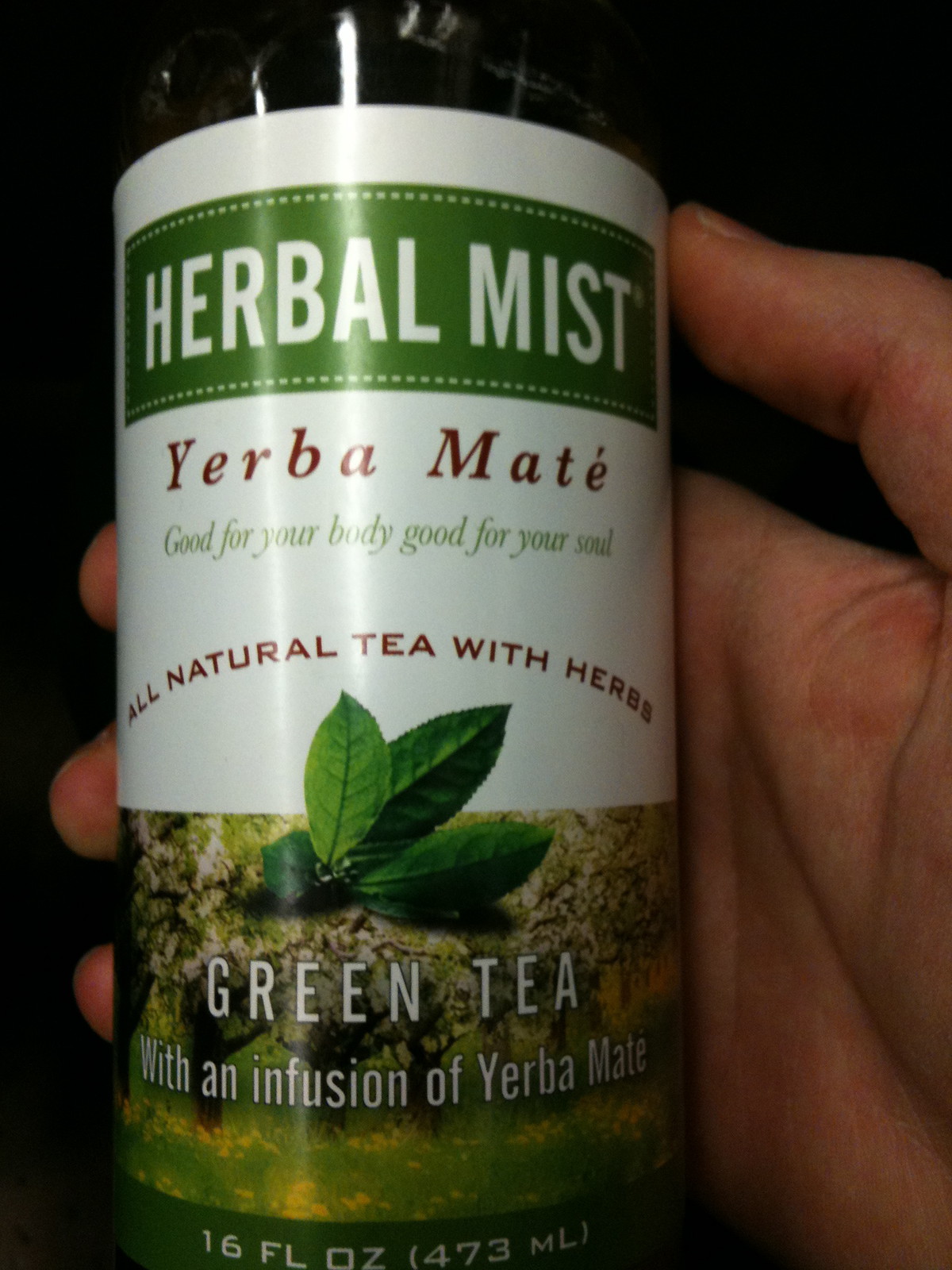The image features a Caucasian hand against a black background, holding a dark-colored bottle with a detailed label. The label has a green banner at the top with bold, white uppercase text that reads "HERBAL MIST." Below this, "Yerba Maté" is written in white letters with an accent on the 'e.' In italicized green text, "Good for your body, good for your soul" is centered below the product name. Further down, in all caps, dark, curved text reads "All Natural Tea with Herbs." The center of the bottle showcases an image of green tea leaves against a tea tree background. In large white text, the bottom of the label states "Green Tea with an Infusion of Yerba Maté." The quantity is noted as "16 FL OZ" and "473 ML" in parentheses.